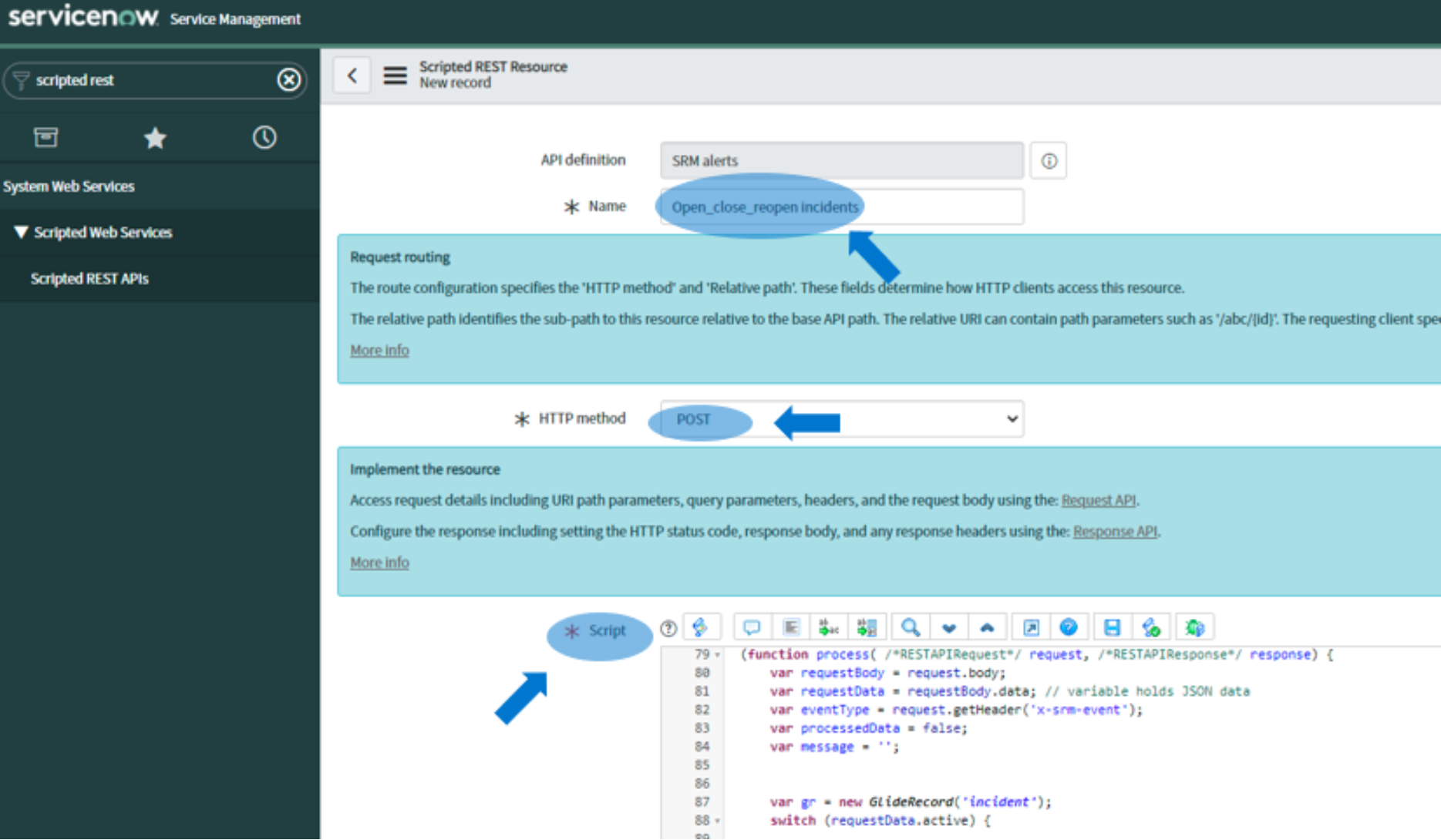**Detailed Descriptive Caption:**

This screenshot captures the interface of the ServiceNow website, specifically focused on service management functionalities. The layout prominently features a left-hand menu shaded in a dark teal color. Near the top of this menu, there is a tag labeled "Scripted REST." 

Across the top of the interface, an inbox icon, a star icon, and a clock icon are visible for navigational purposes. The main content is partitioned into various sections, with a gray bar header displaying "Scripted REST Services" and "New Record." To the left of these headings, there are both a hamburger menu for additional options and a back arrow for navigation.

Underneath the header, one can see a section titled "API Definition" followed by items such as "SRM Alerts," "Name," and "Open_Close_Reopen Incidents," which is highlighted with a blue oval and an accompanying blue arrow pointing at it. 

Further down, a prominent blue rectangle is titled "Request Routing," which provides details about routing configuration, specifying the HTTP method and the relative path.

Below this blue rectangle, a white section specifies "HTTP Method" with "Post" highlighted alongside another blue oval and arrow pointing to it. Another blue rectangle, labeled "Implement the Resource," offers additional information, followed by a detailed area showcasing actual script lines of code. This script section bears a highlighted "Script Title" with an arrow originating from the lower left corner pointing at it, indicating its importance in the scripting process.